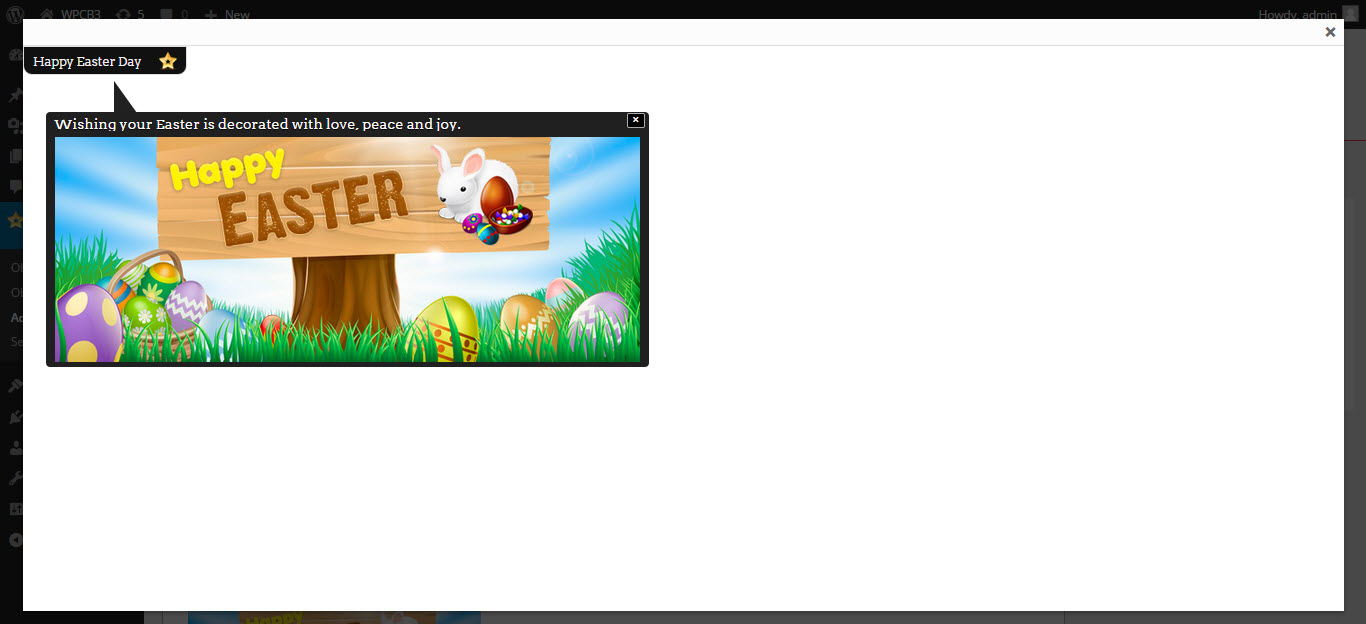The image portrays a large, rectangular monitor screen with a sleek black border. At the top of the screen, there is a bold greeting, "Happy Easter Day." In the upper left-hand corner, a smaller rectangular inset appears, creating a screen-within-a-screen effect. This smaller screen features a slash mark pointing upwards towards the "Happy Easter Day" message.

Within the inset, a black rectangle adorned with a gold star contains a heartfelt message: "Wishing your Easter is decorated with love, peace, and joy." 

The main visual features a whimsical, grassy landscape with a tree trunk emerging from the center. A brown rectangular banner stretches across the top, with the words "Happy Easter" inscribed upon it; "Happy" is highlighted in yellow, while "Easter" is styled in brown. 

Below the banner, a white rabbit adds a playful touch, surrounded by a collection of Easter eggs. Notably, one egg is open, revealing an array of tiny, colorful Easter eggs inside. Nestled in the grass, further brightly decorated foil Easter eggs complete the festive scene.